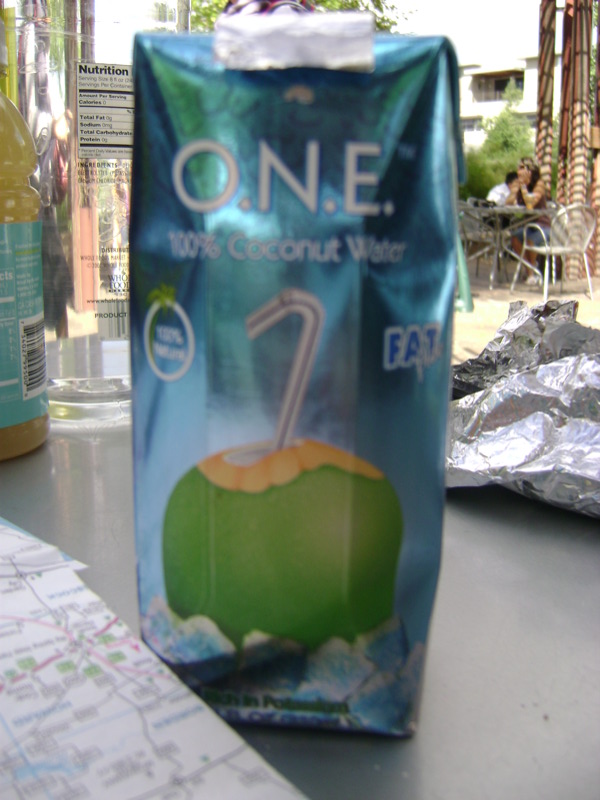The image showcases a mostly-consumed individual-sized carton of ONE brand 100% coconut water, prominently placed on a gray tabletop. The carton, with a blue exterior and an illustration of a green coconut featuring a straw, stands slightly crushed. Surrounding the carton, additional details enrich the scene: to the left side of the coconut water, a drink with a blue label slightly enters the frame, alongside what seems to be a map corner. To the right, a piece of tin foil is visible. In the backdrop, a restaurant setting unfurls with a table and chairs, where a man and a woman are seated. A clear bottle of liquid, possibly water, is seen at the top left corner, merging with the ambient restaurant environment.